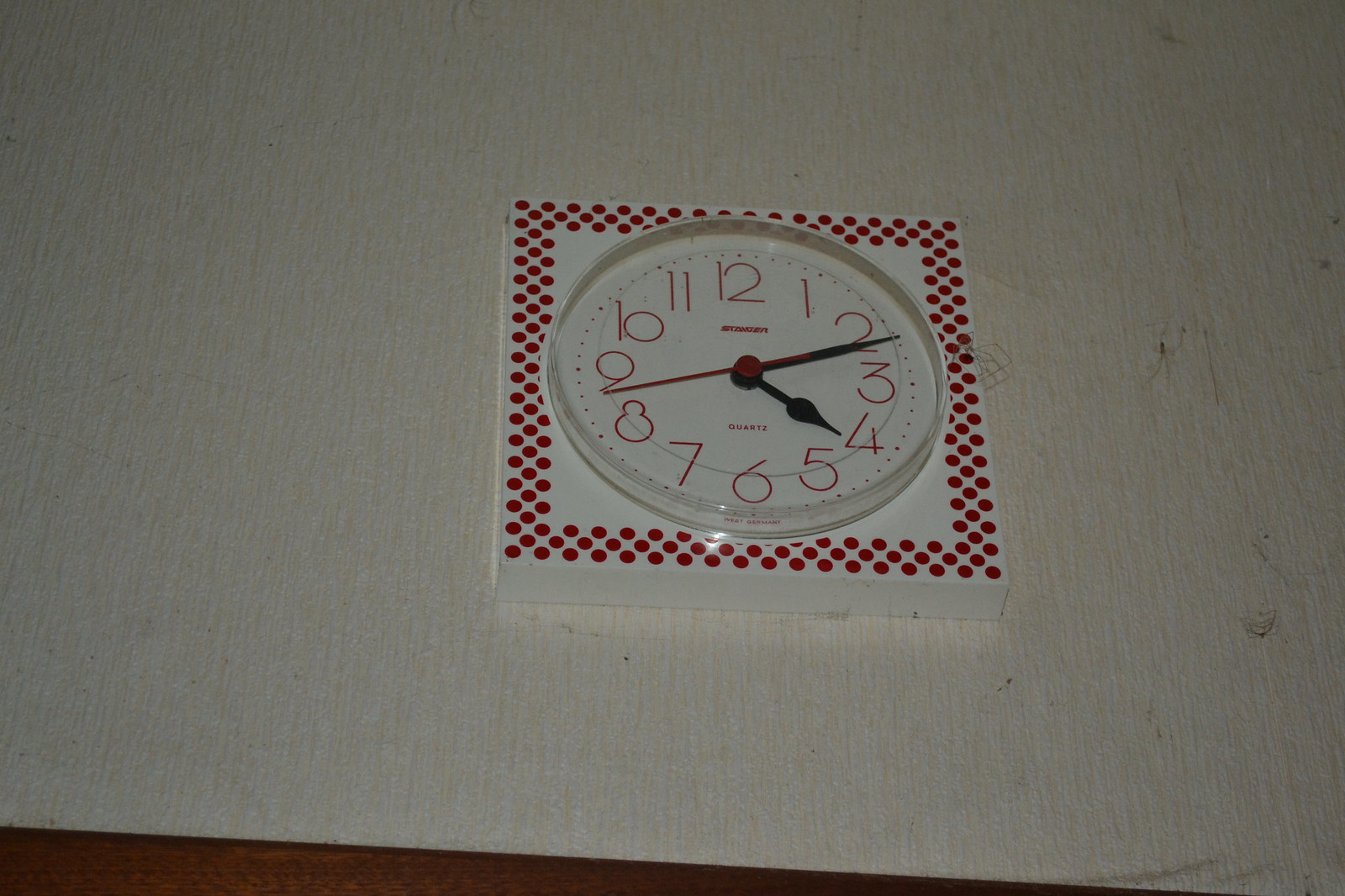This image features a clock mounted on a striking, square, white frame adorned with three rows of evenly spaced, small red circles encircling the edges. The clock itself is round and has a pristine white face. Its timekeeping elements include sleek black hour and minute hands, complemented by a vibrant red second hand, currently positioned between the 8 and the 9, displaying the time as 4:12. The clock's numerals are presented in a contemporary font, enhancing its modern aesthetic. Below the hands, the word "quartz" is prominently printed in red, signifying the type of mechanism within.